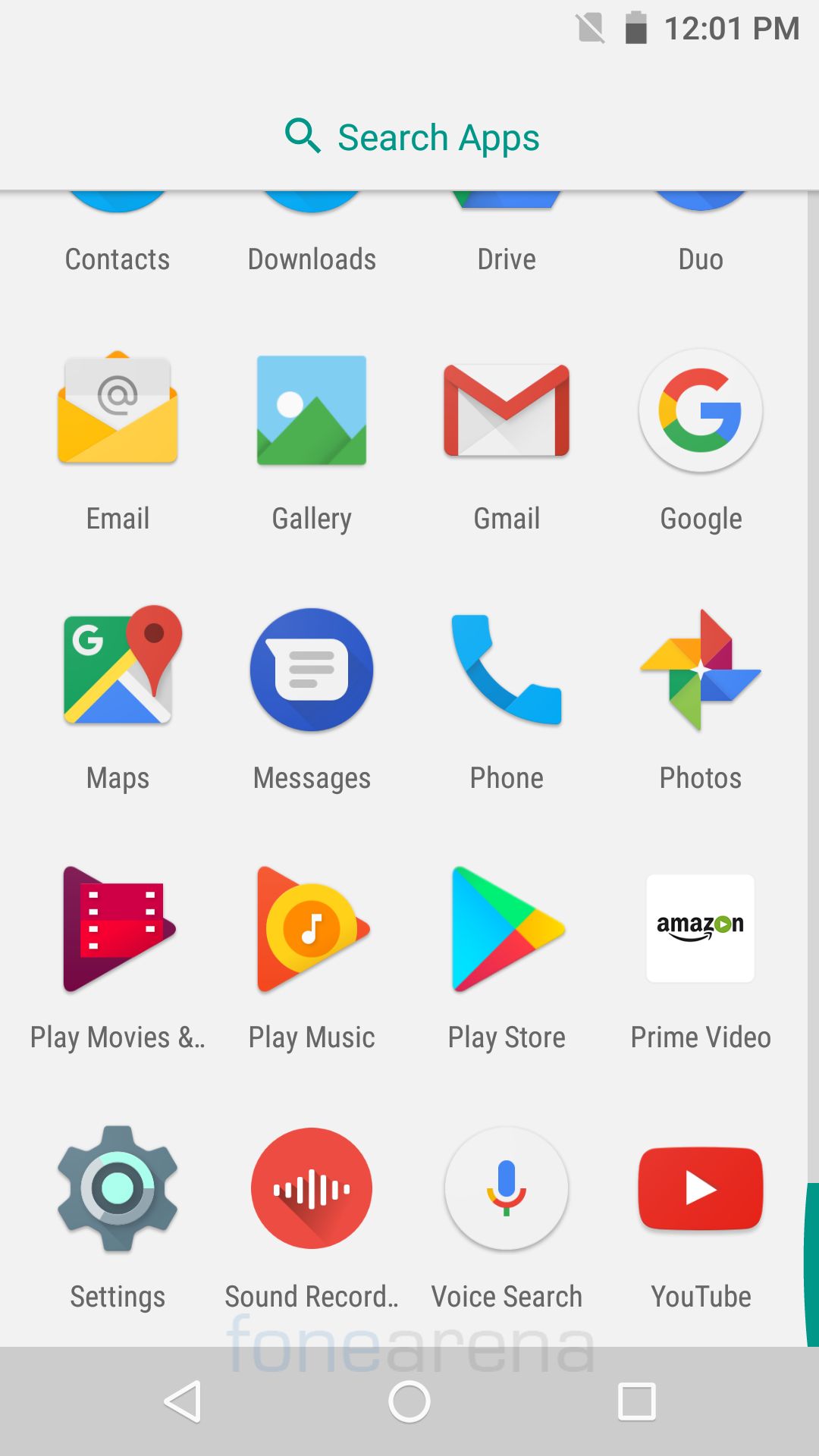This image is a screenshot from a smartphone, illustrating the app drawer interface. At the very top, there’s a prominent white rectangle, partially encasing a teal-colored search bar labeled "Search apps," with a magnifying glass icon to the left of the text. The status bar at the top right corner shows a battery indicator and the time, which is 12:01 p.m.

Within the main portion of the screen, apps are meticulously organized into a grid of four columns by five rows, ensuring an even layout. This grid showcases various app icons, each distinctly representing its respective application. The visible apps are:
- **Top Row (cut off):** Contacts, Downloads, Drive, Duo.
- **Second Row:** Email, Gallery, Gmail, Google.
- **Third Row:** Maps, Messages, Phone, Photos.
- **Fourth Row:** Play Movies, Play Music, Play Store, Prime Video.
- **Fifth Row:** Settings, Sound Recording, Voice Search, YouTube.

Near the bottom, there’s a semi-transparent horizontal gray menu bar, displaying three navigation icons: a left-pointing arrow for 'Back', a circle for 'Home', and a square for 'Recent Apps.'

On the right side of the screen, a vertical scroll bar is visible. The scrollbar's position indicates that the user has scrolled all the way down as evidenced by the solid blue section at the bottom of the thin gray scroll indicator.

Each app icon is clearly defined with its associated graphic, providing a visual representation of the app's purpose or brand.